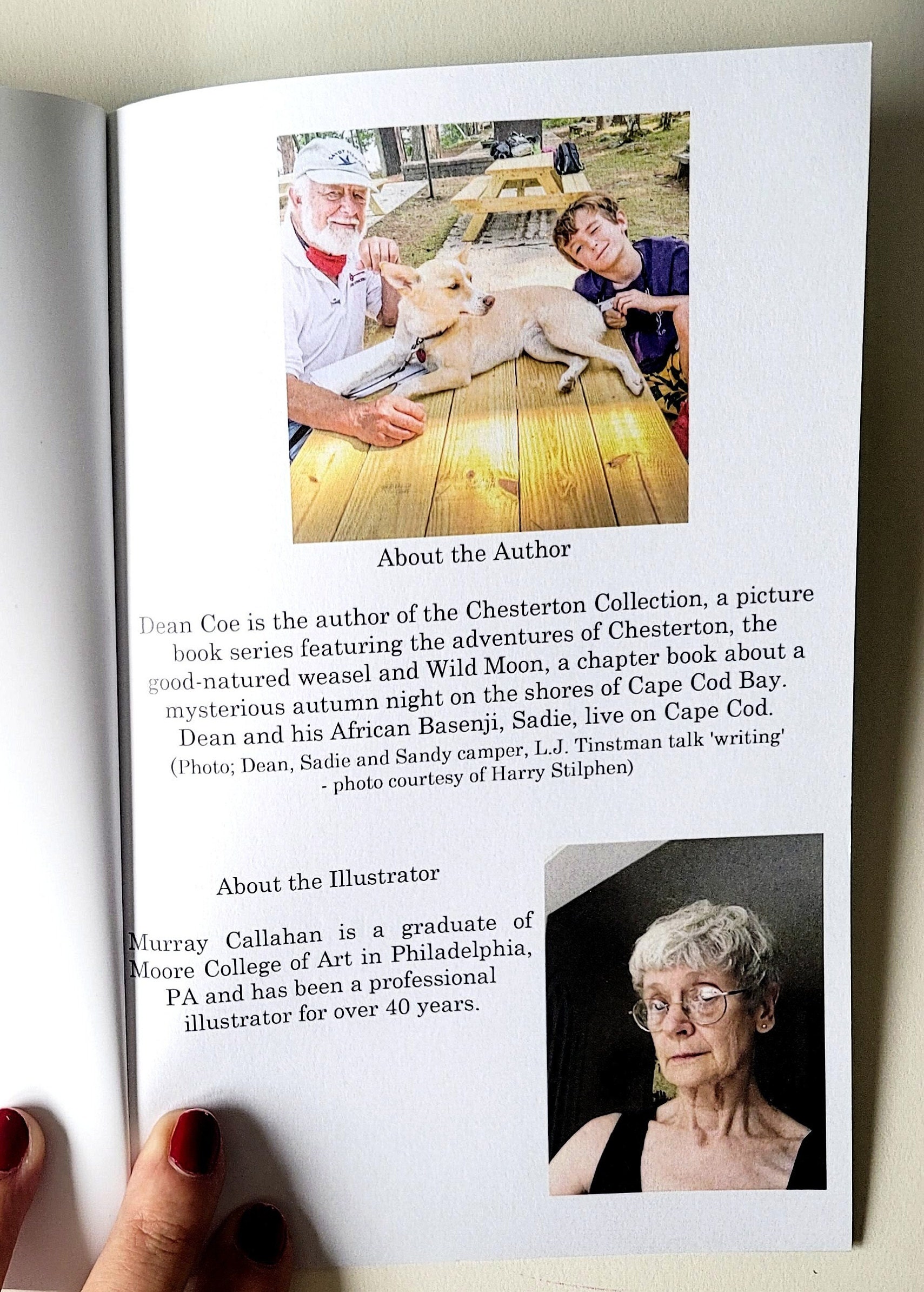This open page of a book features two key sections: "About the Author" and "About the Illustrator." At the top, a photograph captures an older gentleman and a young boy seated at a picnic table with a small tan dog positioned between them. The older gentleman sports a white collared shirt over a red undershirt, a white hat adorned with a blue bird, and a white beard. The young boy to his right is dressed in a blue t-shirt and yellow and black shorts, with brown hair visible. Another empty picnic table is situated in the background. The accompanying text identifies the author as Dean Coe, known for the "Chesterton Collection," a picture book series about the adventures of Chesterton, a good-natured weasel, and "Wild Moon," a chapter book about a mysterious autumn night on the shores of Cape Cod Bay. Dean resides on Cape Cod with his African Basenji, Sadie. Below this, the "About the Illustrator" section introduces Murray Callahan, who graduated from Moore College of Art in Philadelphia, Pennsylvania, and has been a professional illustrator for over 40 years. A photograph of Callahan depicts her with short gray hair, large circular bifocals, wearing a black tank top, against a white and black background. The photo captures a woman's hand, adorned with red nail polish, holding the book open.